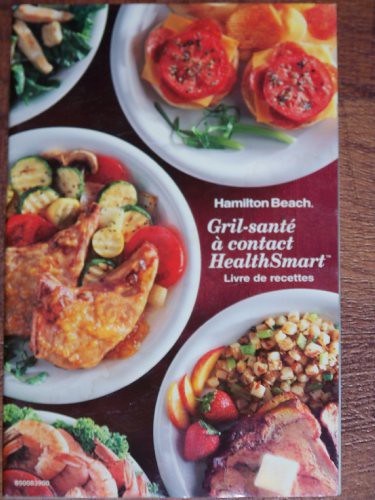This is a high-resolution, color photograph taken from a top-down angle, showcasing the cover of a manual. The cover is vibrant and prominently features the text "Hamilton Beach, Grille Santé, Contact HealthSmart, Livre de Recettes." The cover is adorned with an array of appetizing dishes. 

In the top right corner, a round white plate holds an artful arrangement of tomatoes atop cheese. To the left, spilling out of the frame, is a fresh salad composed of crisp lettuce leaves and tender chicken pieces. Directly beneath the salad, another white plate showcases a hearty meal of chicken served alongside roasted vegetables, including zucchini and tomatoes. 

Partially visible in the bottom left corner, a bed of lettuce cradles a generous portion of shrimp. On the right side of the cover, another white plate, also partially out of frame, displays a wholesome breakfast spread featuring toast layered with butter, neatly chopped potatoes, apple slices, and two whole strawberries. The composition of the food on the cover is both appealing and expertly arranged, highlighting the culinary delights to be found within the manual.